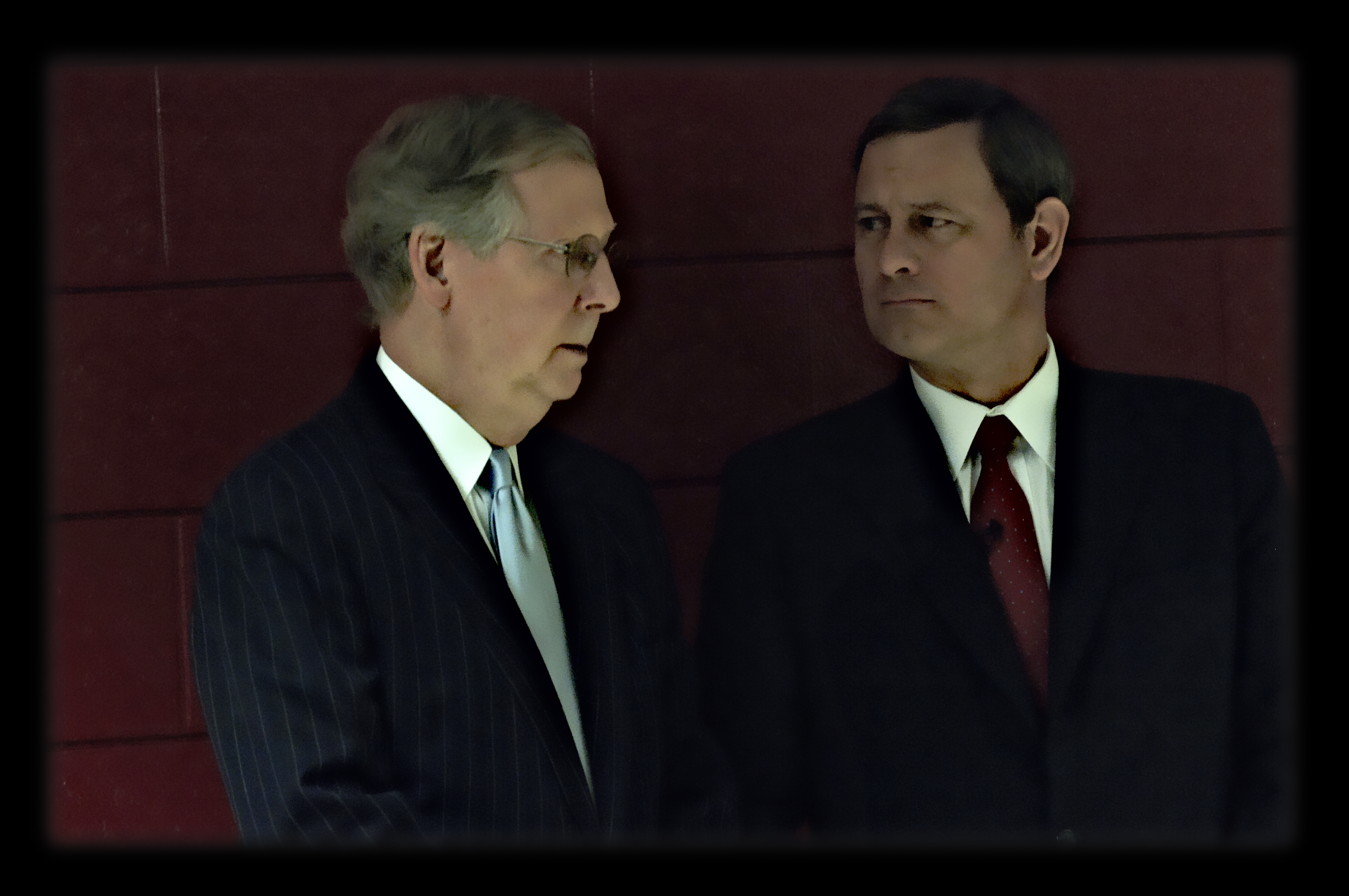In the image, two men are standing next to each other in conversation, dressed in formal attire. The man on the left, who resembles Senator Mitch McConnell, is wearing a dark pinstripe suit with a white dress shirt and a light blue tie. He has gray hair, glasses, and appears to be in his 60s. His mouth is slightly open as if he is speaking. The man next to him is younger, likely in his late 40s, with short dark hair and clean-shaven. He is dressed in a black suit jacket, white dress shirt, and a cranberry-colored tie. This man is looking attentively at the older gentleman. Behind them is a block wall painted a dark burgundy or purple hue, influenced by the lighting in the scene.